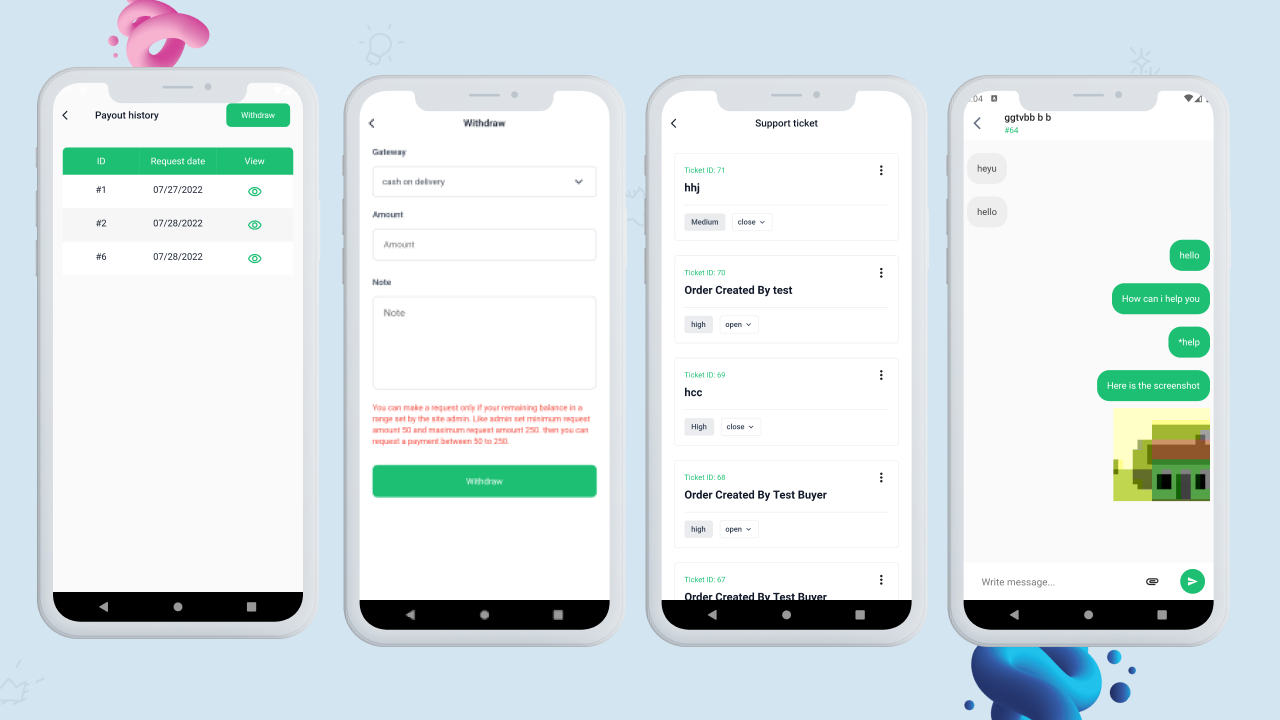The image features a light blue background showcasing four smartphone screenshots arranged horizontally. A pink three-dimensional coil with small accompanying dots floats above the top left smartphone. Each screenshot displays distinct app interfaces:

1. The top left screen displays a "Payout History" section featuring a green "Withdraw" button on the right. Below the button, there's a table with columns labeled "Number ID," "Request Date," and "View," displaying respective IDs, dates, and eye icons for viewing details.
 
2. The second screen from the left is titled "Withdraw." It includes fields and options for "Gateway" (with "Cash on Delivery" noted), "Amount," and "Notes." The interface features some red text for alerts or instructions and a green "Withdraw" button for submitting requests.

3. The third screenshot focuses on "Support Ticket" information. It lists a "Ticket ID," annotated as "HHJ," along with details such as "Order Created by Test." It also includes buttons for prioritizing support requests (e.g., marking them high or low priority).

4. The far right screen resembles a text conversation interface, displaying gray message bubbles on the left and green bubbles on the right, indicative of a chat format. Additionally, there's a picture of a house within the chat conversation.

Below the far right smartphone, a blue 3D coil similar to the pink one can be observed, enhancing the visual balance of the composition.